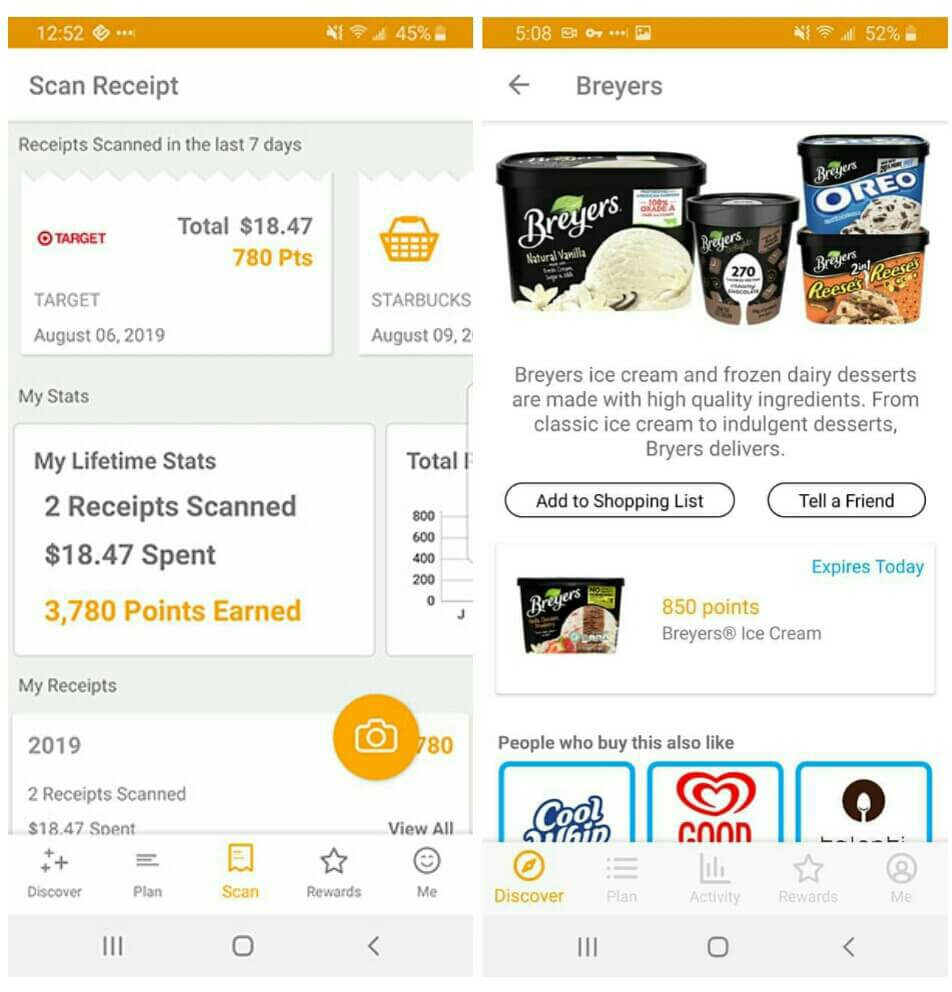The image features two side-by-side screenshots captured from a cell phone, each adorned with a yellow banner at the top.

**Left Screenshot:**
- The time displayed is 12:52.
- The top right corner shows several white icons: notifications off, Wi-Fi on, full signal bars, and a battery at 45%.
- Below, a white box features the word "Target" in red, with a total of $18.47 in gray text.
- Underneath, in yellow text, it reads "780 points" with the date "August 6, 2019."
- Another white box below details "My lifetime stats" in gray text: "Two receipts scanned," "$18.47 spent," and "3,780 points earned" highlighted in yellow.

**Right Screenshot:**
- Displays images of Breyers ice cream in four distinct flavors: vanilla, chocolate, Oreo, and Reese's Pieces.
- There are two interactive buttons beneath the images: "Add to shopping list" and "Tell a friend."

Overall, the detailed layout of the screenshots highlights the user's spending and rewards points with clear, easy-to-read information and visual elements for added context.